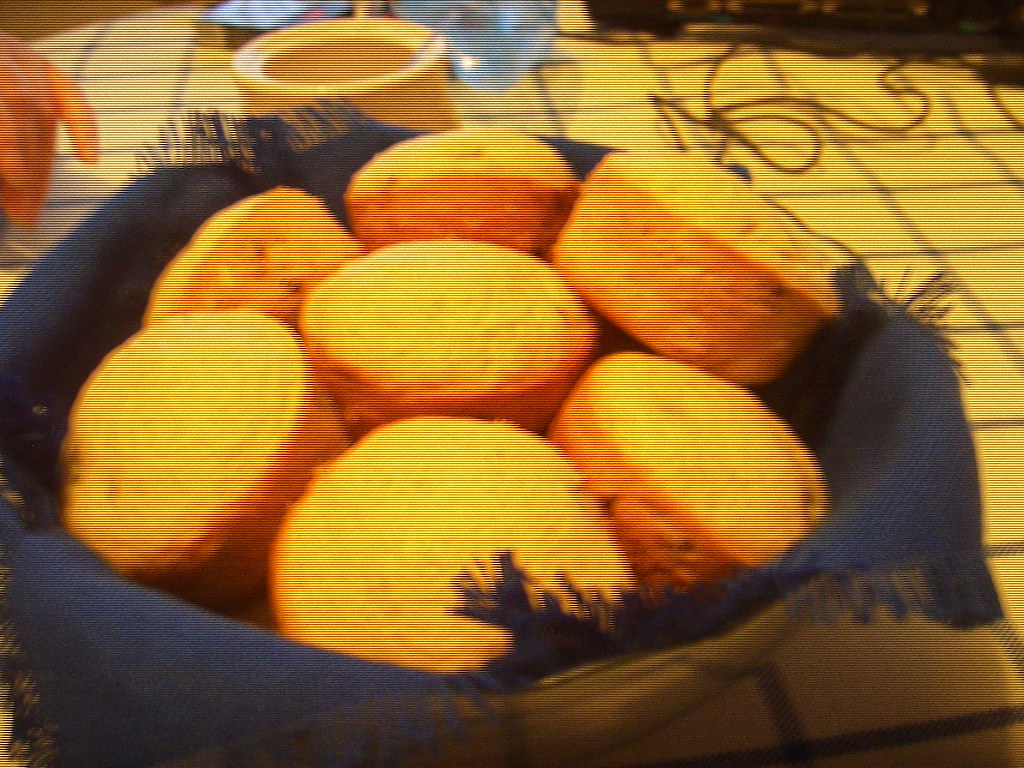This slightly out-of-focus photograph features a close-up of seven or eight small, round cornbread muffins nestled in a basket, detailed with a dark blue, fringed napkin. The basket itself, made from a light blonde wicker material, rests on a table with a yellow, broadly checked tablecloth intersected by blue lines. Adding to the homey atmosphere, a cup of coffee and a human hand are visible in the background, providing a sense of scale and context. The table also holds a few miscellaneous items and cables, suggesting a cozy, lived-in scene. The image appears to have significant color banding or streaking, reminiscent of issues seen with old CRT screens or ink problems in printers, especially notable with the yellow streaks running through the muffins and the fabric, yet the blue napkin and darker elements remain largely unaffected.